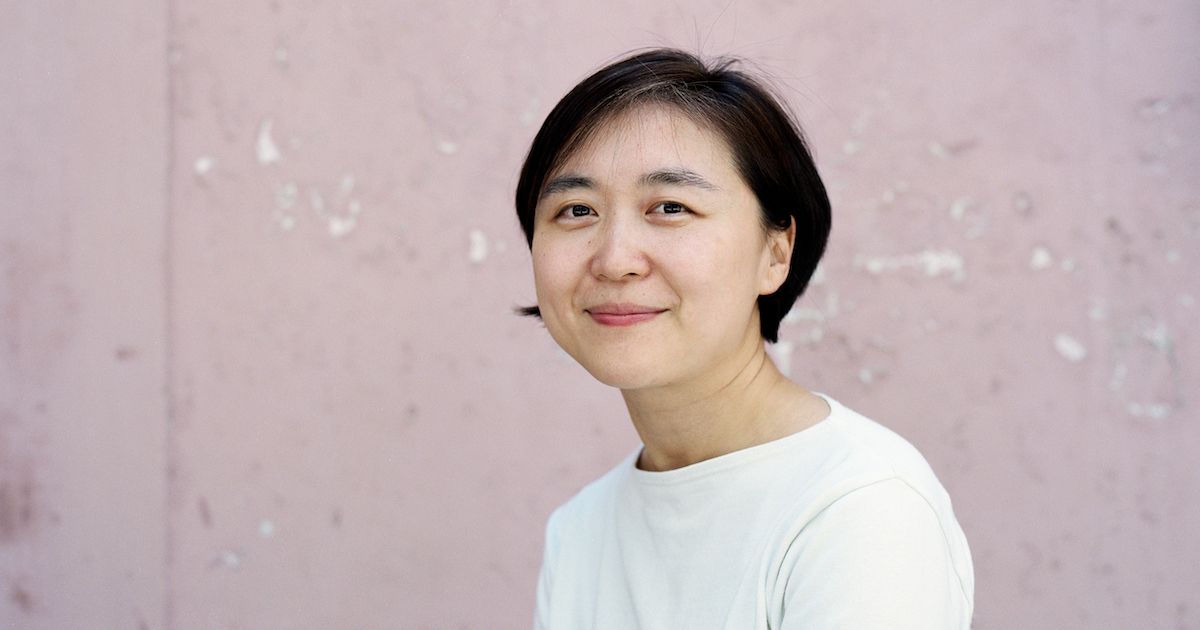This is a detailed color headshot of an Asian woman who appears to be middle-aged. She is wearing a plain white shirt and has short, black hair that extends just past her ears. Her hair is parted slightly to the side and brushed back from her ears. She is smiling gently without revealing her teeth. She has black eyebrows and dark eyes, and no visible jewelry. The woman is almost perfectly centered in the photo, with her upper arms and head visible. She is facing the camera at a slight angle, around 45 degrees. The backdrop is a pinkish, weathered wall with areas where the paint has peeled, revealing white patches beneath. The background is blurred out to keep the focus on her.